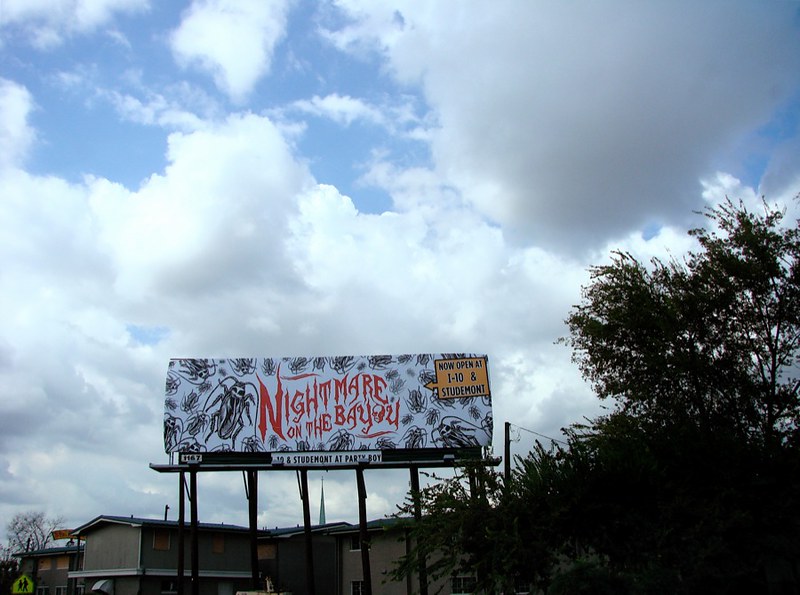The image is a horizontally rectangular photograph taken from a ground perspective looking up towards the sky. Dominating the upper region of the background are expansive, puffy white clouds set against a pale blue sky. Moving down towards the lower portion of the frame, on the right side, a dense cluster of trees and shrubs appears, shrouded in shadow and therefore lacking discernible colors. Spanning horizontally along the bottom edge of the image, the top of a building is visible. Positioned in the foreground above the building is a large billboard. The billboard's background is white and adorned with various black illustrations of bugs. Bold red text at the center of the billboard reads, "Nightmare on the Bayou."